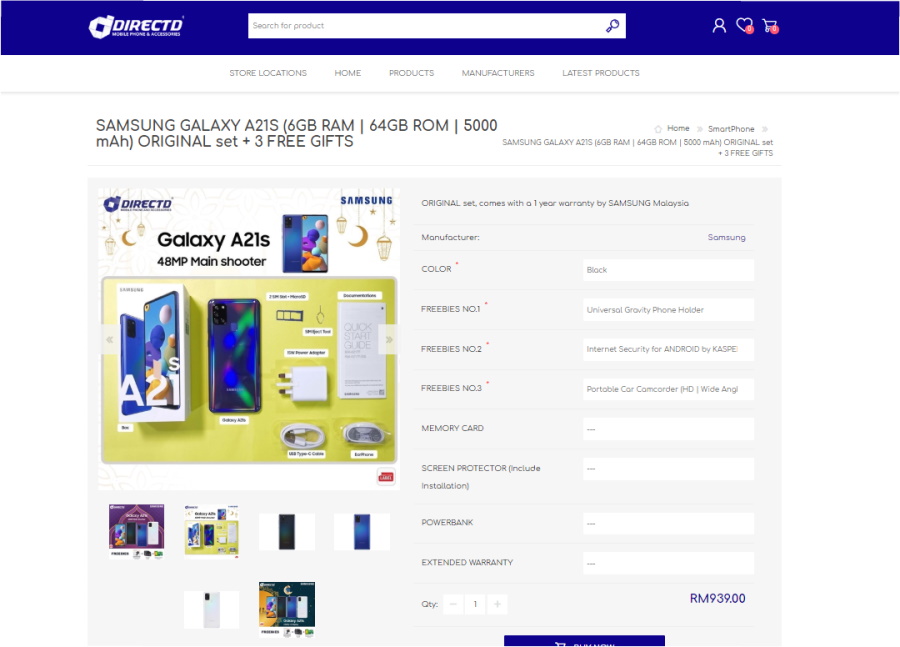At the top of the screen, a purple border with the text “DirectD” is accompanied by the tagline “Mobile Phone and Accessories” and a white D logo. Adjacent to this is a white search bar displaying the prompt “search for product” with a magnifying glass icon on the right. Further along the top, icons for a user profile, a wishlist (heart), and a shopping cart are present. Below these, navigation options include “Store Locations,” “Home,” “Products,” “Manufacturers,” and “Latest Products.”

The primary content focuses on the Samsung Galaxy A21s. The details highlight the device’s 6GB RAM, 64GB ROM, and a 5000 mAh battery, along with a promotion offering three free gifts with the original set. The product path is laid out as “Home > Smartphone > Samsung Galaxy A21s.”

A prominent image showcases the DirectD Galaxy A21s. The device is featured with a 48-megapixel main camera. The background of the image is gold-colored, and prominently displays a white box containing the phone, with the phone itself, the charger, cables, and other included items laid out.

On the right side of the screen, several menus provide additional information: 

- **Manufacturer:** Samsung 
- **Color:** Black 
- **Freebies:** 
  1. Universal Gravity Phone Holder 
  2. Internet Security for Android 
  3. Portable Car Camcorder with HD wide-angle capability